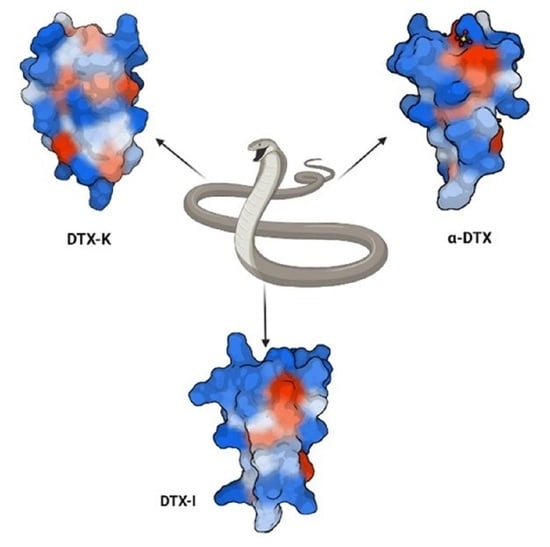The diagram features an artistic black-and-white illustration of a snake, likely a cobra, centrally positioned. Surrounding the snake are three distinct black arrows pointing away from its body: one near the head, one near the midsection, and one near the tail tip. Each arrow directs attention to colored, three-dimensional genetic diagrams that are labeled with different neurotoxins associated with snake venom. The upper left arrow points to DTX-K, the arrow to the right highlights alpha DTX (A-DTX), and the bottom arrow indicates DTX-I (DTX-1). The colorful diagrams in blue, white, and red signify the genetic makeup of these neurotoxins, specifically targeting voltage-gated potassium channels, emphasizing their potential use and study in various fields.